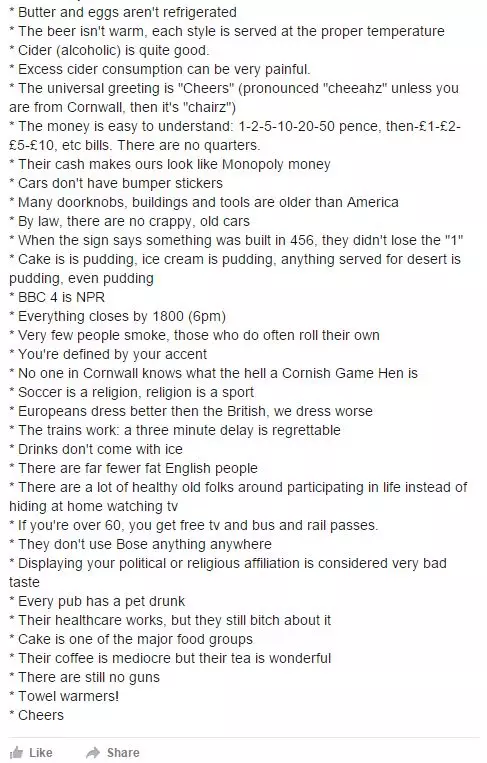**A Tourist's Observations from Cornwall:**

- Butter and eggs are not refrigerated.
- Beer is served at the proper temperature for each style.
- Alcoholic cider is quite good but can be painful if consumed in excess.
- The universal greeting is "cheers," pronounced "chairs" unless you are from Cornwall.
- The money system is simple: 1, 2, 5, 10, 20, and 50 pence, followed by 1, 2, 5, and 10-pound notes. There are no quarters, and their cash makes American dollars look like Monopoly money.
- Cars do not have bumper stickers.
- Numerous doorknobs, buildings, and tools are older than America.
- By law, old dilapidated cars are not allowed.
- Historical dates are true, like when a sign says something was built in 456, it wasn’t a typo.
- Dessert is referred to as pudding, regardless of whether it is cake, ice cream, or actual pudding.
- BBC 4 is the equivalent of NPR.
- Everything closes by 6 PM (1800 hours).
- Few people smoke, but those who do often roll their own cigarettes.
- No one in Cornwall knows what a Cornish game hen is.

These details capture the quirky and unique aspects of visiting Cornwall from an American tourist’s perspective.